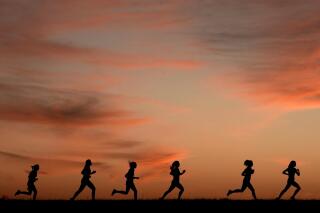In this dynamic photograph, six individuals, seemingly female, are captured in mid-run at either sunrise or sunset. They form striking black silhouettes against the horizon, making it impossible to discern specific details about them other than their hair bouncing in the wind. They are racing from left to right across a stretch of level land, possibly dirt, track, or beach, which is also silhouetted and appears flat with no hills or undulations. 

The sky behind them is a breathtaking array of pink, purple, and blue tones, highlighted by wispy clouds that reflect the vivid colors of the rising or setting sun. The sun itself is no longer visible, casting an ethereal glow that paints the scene with a serene yet energetic ambiance.